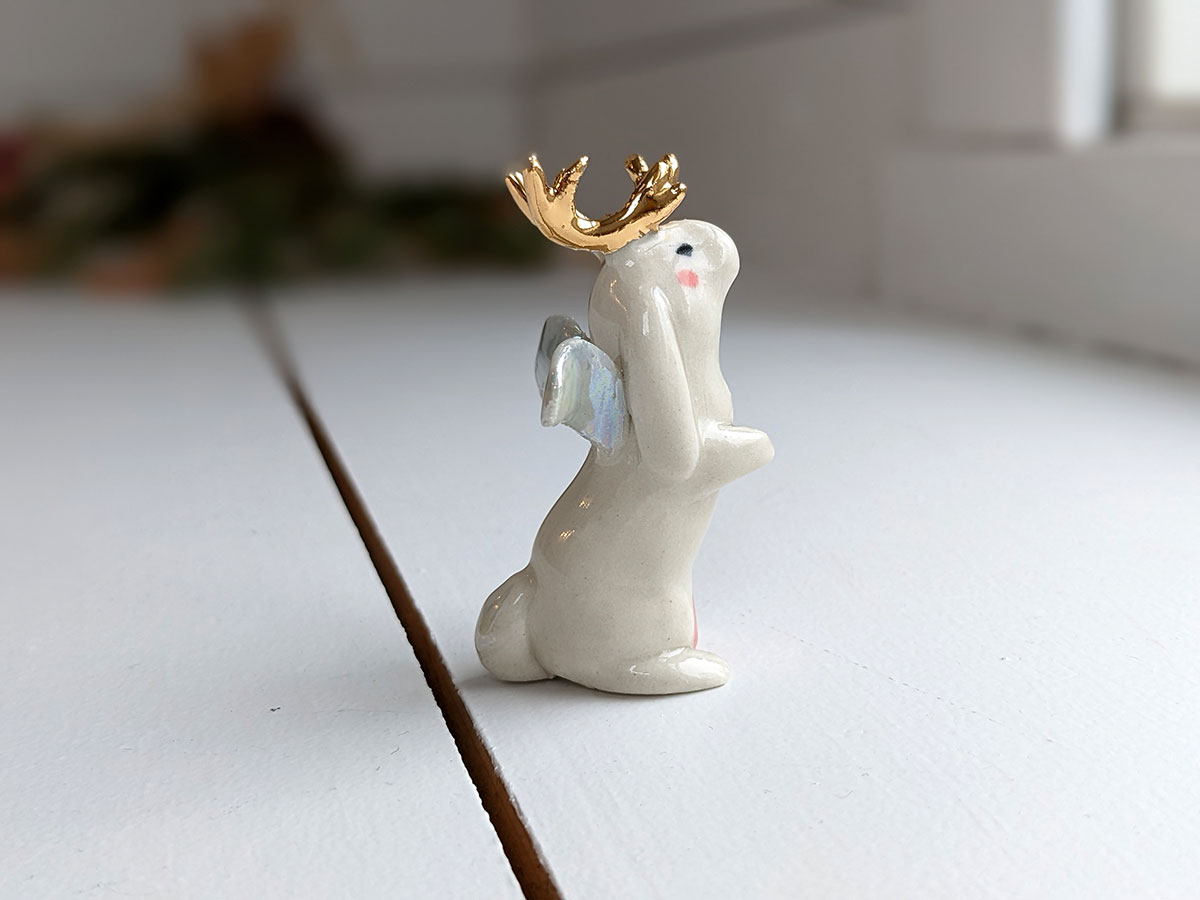The image features a detailed close-up of a small ceramic figurine depicting a white rabbit. The rabbit, with one front paw and one back paw visible, is sitting upright on a white, snow-painted wooden surface that has visible slabs and a crack down the middle. The rabbit has long ears, a black eye, and a small pink mark on its cheek. It is adorned with golden antlers on its head and silver wings on its back, giving it a whimsical appearance. The figurine's posture, with its paws out in front as if praying, adds a charming touch. In the background, to the right, there’s a window ledge, and to the left, there are some blurry dark figures, enhancing the bright, ethereal quality of the overall scene.